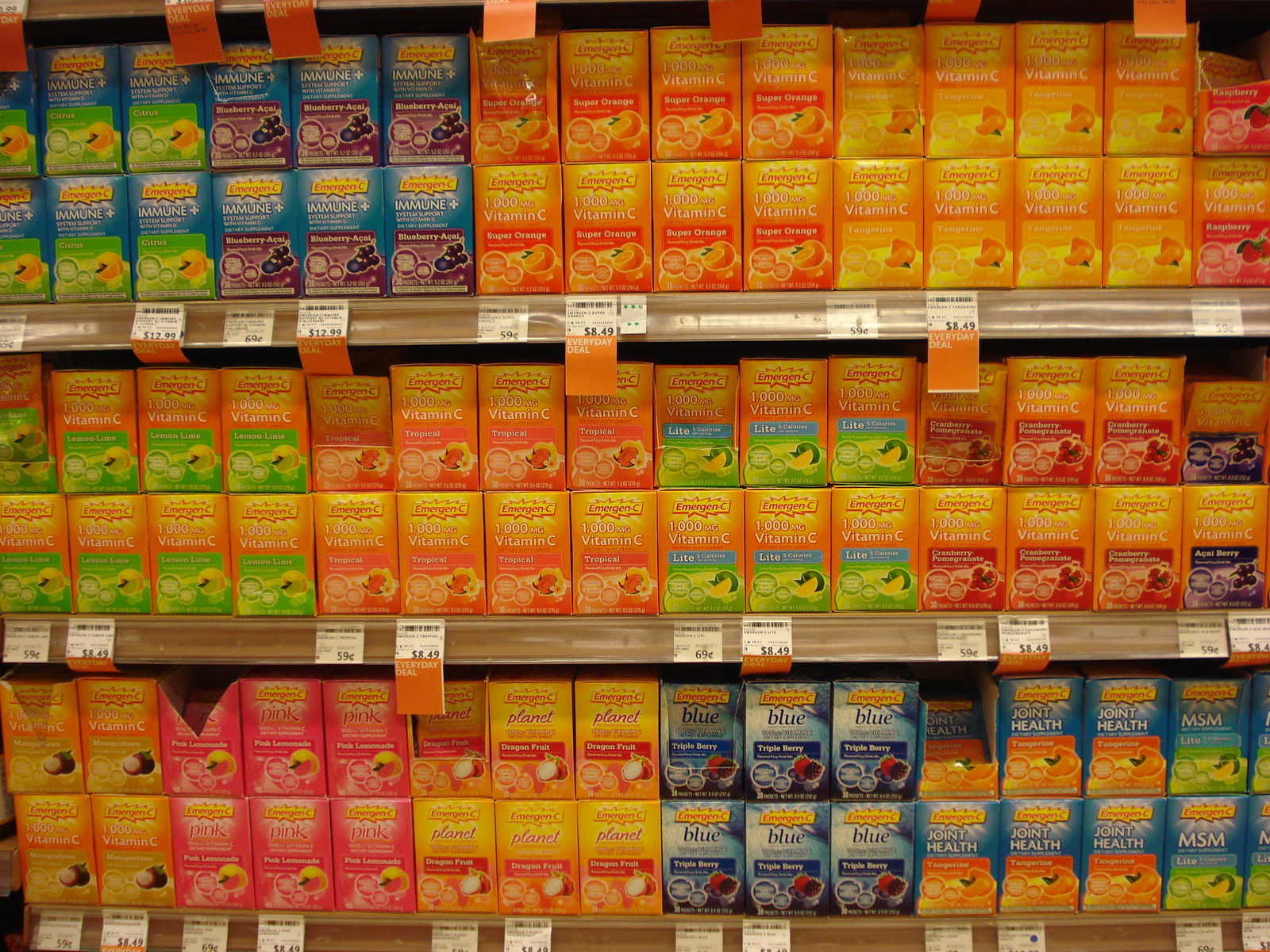This image captures a well-stocked grocery store aisle featuring three packed shelves of various Emergency Vitamin C supplements. The shelves are lined with a vibrant array of brightly colored boxes, predominantly in hues of orange, red, blue, and green. Each box contains powdered health drinks aimed at promoting wellness, available in different flavors and specialized formulas. Notable varieties include Emergency Immune Plus with citrus and elderberry flavors, the 1000mg Vitamin C Super Orange, and formulations targeting specific health concerns such as joint health with MSM. The prices range from $8.49 to $12.99, with some items marked as "Everyday Deal," indicating a discount. The organized display includes clear white and orange tags for easy price identification. Overall, the image showcases the brand's extensive lineup of vitamin supplements designed to cater to various health needs.